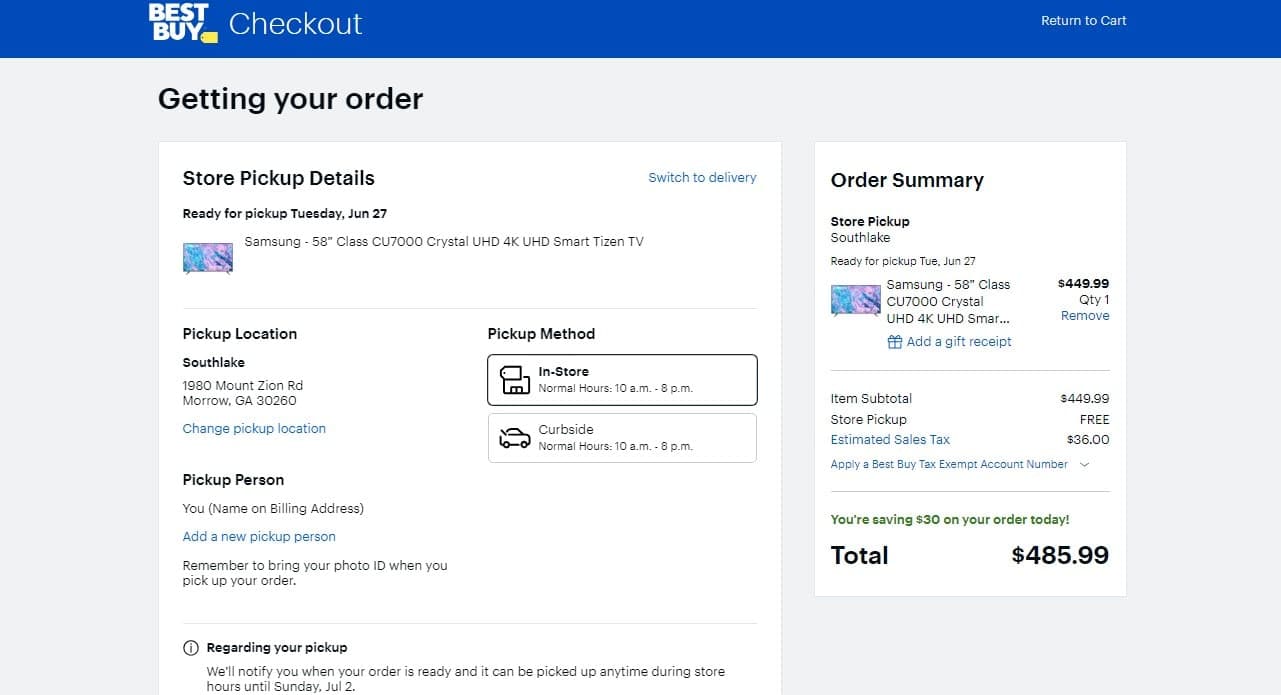Screenshot of a Best Buy Checkout Page for Samsung 58-Inch Crystal UHD Smart TV

The screenshot displays a Best Buy checkout page with a prominent blue header row at the top, featuring the Best Buy logo on the top left alongside the label "Checkout." On the top right, a link reads "Return to Cart." Below the header, the page title states "Getting Your Order."

On the left side, a section provides store pickup details. The item for pickup is a Samsung 58-inch Class CU7000 Crystal UHD 4K UHD Smart Tizen TV, scheduled for Tuesday, June 27th. The pickup location is at Southlake, 1980 Mount Zion Road, Morrow, Georgia 30260, with an option to change the pickup location via a link. The section also includes fields for the pickup person, though no name or billing address is listed. Customers can choose a pickup method, either in-store or curbside.

On the right side, the order summary is displayed. It reiterates the store pickup details, confirming the Samsung TV's availability for pickup on Tuesday, June 27th. Users have the option to add a gift receipt or remove the item from their cart. The price of the TV is listed at $449.99, with a quantity of one. The item subtotal matches the price at $449.99, with free store pickup. Estimated sales tax amounts to $36. The page provides an option to apply a Best Buy tax exempt account number. A note indicates a $30 savings on the order, bringing the total to $485.99.